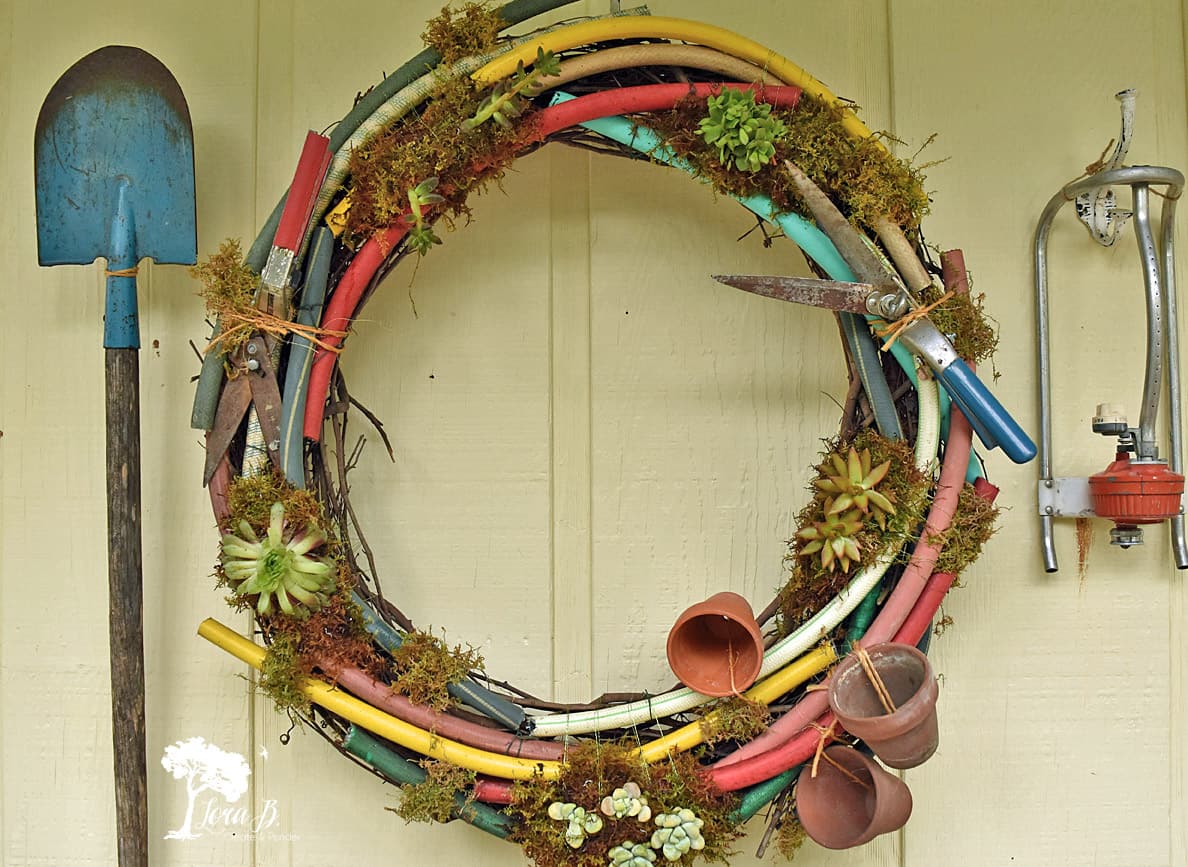This image captures a whimsical and artistic garden decoration set against a butter-colored plank wall, reminiscent of barn siding. Central to the composition is an inventive wreath crafted from various segments of garden hoses, each cut into approximately 12-inch lengths. The hoses come in a vibrant array of colors, including red, yellow, pink, green, white, and black, forming a complete circle. The voids of the hoses are filled with moss and succulents, lending a lush, green appearance to the wreath.

At the bottom right of the wreath, there's a charming arrangement of three small terracotta pots. Nestled among the elements are two pairs of old gardening shears: one with red handles on the left and another with blue handles on the right. On the right-hand side of the wall, hanging on a hook, is an antique silver lawn sprinkler, possibly from the 1950s or 60s, featuring a distinctive old-time fan-shaped design for watering.

To the left of the wreath is a well-worn blue shovel with a patina’d wooden handle. The shovel’s handle shows significant weathering, indicative of many seasons of use. Additionally, the bottom left-hand corner of the image includes a white tree with the inscription "Laura B." and some smaller, unreadable letters below. This entire assembly celebrates the creativity and resourcefulness of repurposing everyday gardening tools into a vibrant, earthy piece of garden art.